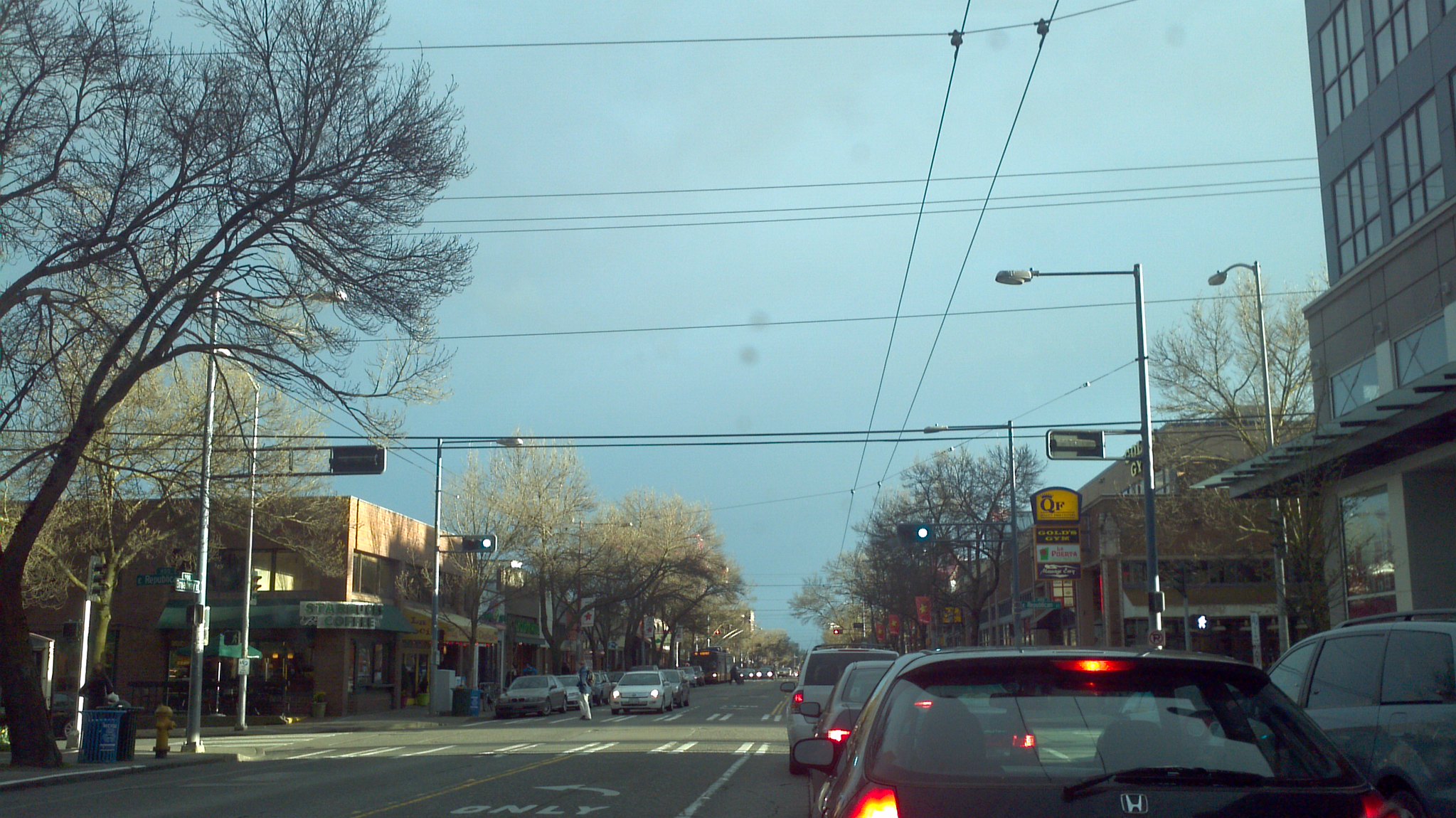This image captures a scene from inside a car at an intersection in a small town or city. The driver appears to be positioned at a stoplight, with the light currently green. In front of the vehicle, there's a line of at least three cars, including a noticeable black Honda. On the opposite side, there's oncoming traffic and a silver vehicle attempting to merge into the lane, with a car behind it showing brake lights, possibly to let it in.

To the left, there's a dedicated left-turn lane. Various one-story buildings that house businesses, including a Gold's Gym and a Starbucks Coffee on the corner, flank the intersection. A person is visible crossing the street in the pedestrian lane, and further back, a bus is parked close to the curb. The sky is blue with several power lines and streetlights crisscrossing above. Leafless trees, indicative of winter, line the street, and some have hints of budding flowers, suggesting they may produce pollen.